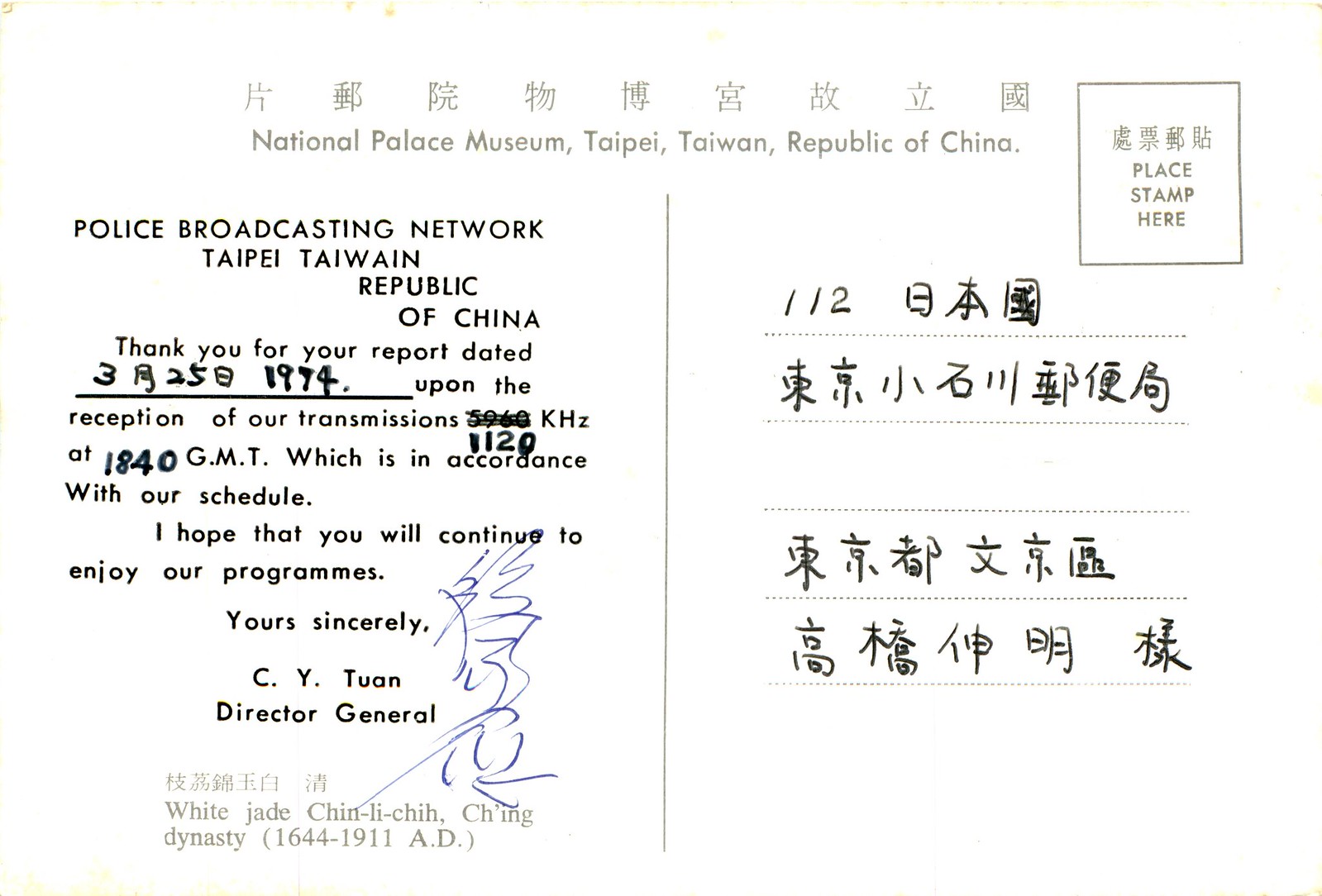This detailed image depicts a historically significant postcard displayed in the National Palace Museum, Taipei, Taiwan, Republic of China. At the top of the postcard, traditional Chinese characters indicate its association with the museum. To the top right, there's a vertically oriented rectangle with four Chinese characters, followed by an English translation instructing, "Please stand here." The postcard's left side is prominently marked with "Police Broadcasting Network, Taipei, Taiwan, Republic of China." The main text expresses gratitude for a report dated March 25th, 1974, concerning the reception of their transmissions on 1128 kilohertz at 1840 GMT, confirming it matches their broadcast schedule. The card conveys the senders' hopes that the recipient continues to enjoy their programs. It is signed, "Yours sincerely, C.Y. Tuan," identified as the Director General, accompanied by his signature on a subtle white background.